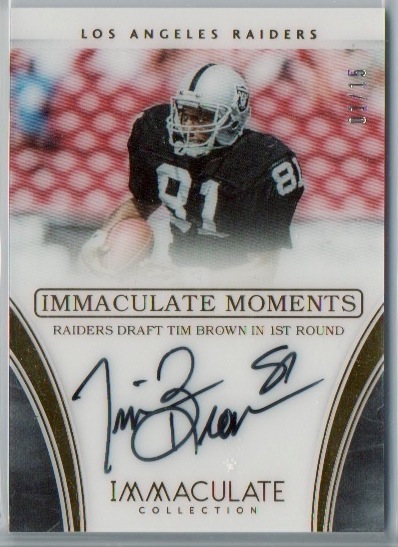This detailed image is a high-end collector's item featuring the Los Angeles Raiders, highlighted by the inscription "Immaculate Moments Raiders draft Tim Brown in first round," and is signed by Tim Brown in black ink. The card, set against a blurry stadium with indistinct red seats in the background, captures Tim Brown in action. He is depicted wearing a silver helmet with a black stripe and a black jersey bearing the number 81, as he holds a football and runs towards the left. The top of the card prominently displays "Los Angeles Raiders" in black text on a white bar. The bottom section, framed by a gray border with rounded edges featuring brown stripes, bears the signature and reads "Immaculate Collection," solidifying its status as a unique and artistic piece of memorabilia.